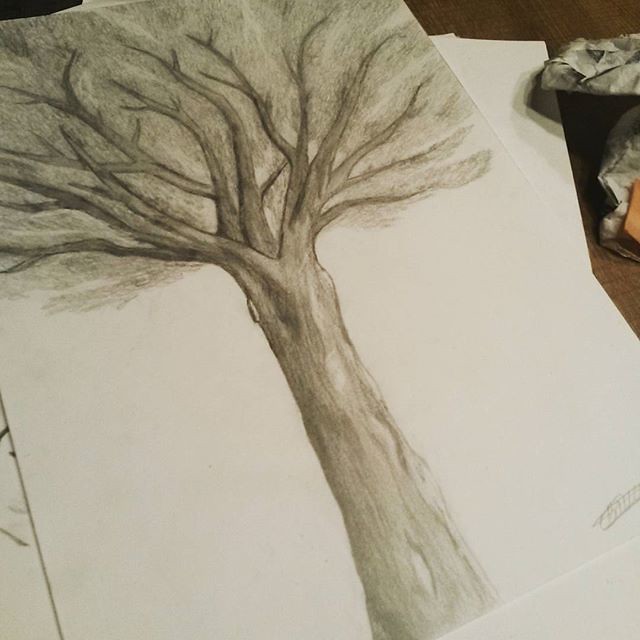A detailed and lifelike pencil (possibly charcoal) drawing of a large oak tree is prominently displayed on a piece of white sketchbook paper. The sketch, approximately 8.5 by 11 inches in size, features a robust, elongated trunk with vivid, naturalistic branches extending upward. The tree's canopy, suggested by gray, feathered shading, adds depth although it remains somewhat abstract compared to the finely detailed trunk and branches. In the lower right-hand corner of the drawing, the artist's signature is visible. The paper lies at a slight left-to-right diagonal angle, resting atop several other sheets. In the upper right-hand corner, a dirty tissue, likely used for smudging, hints at the drawing process.